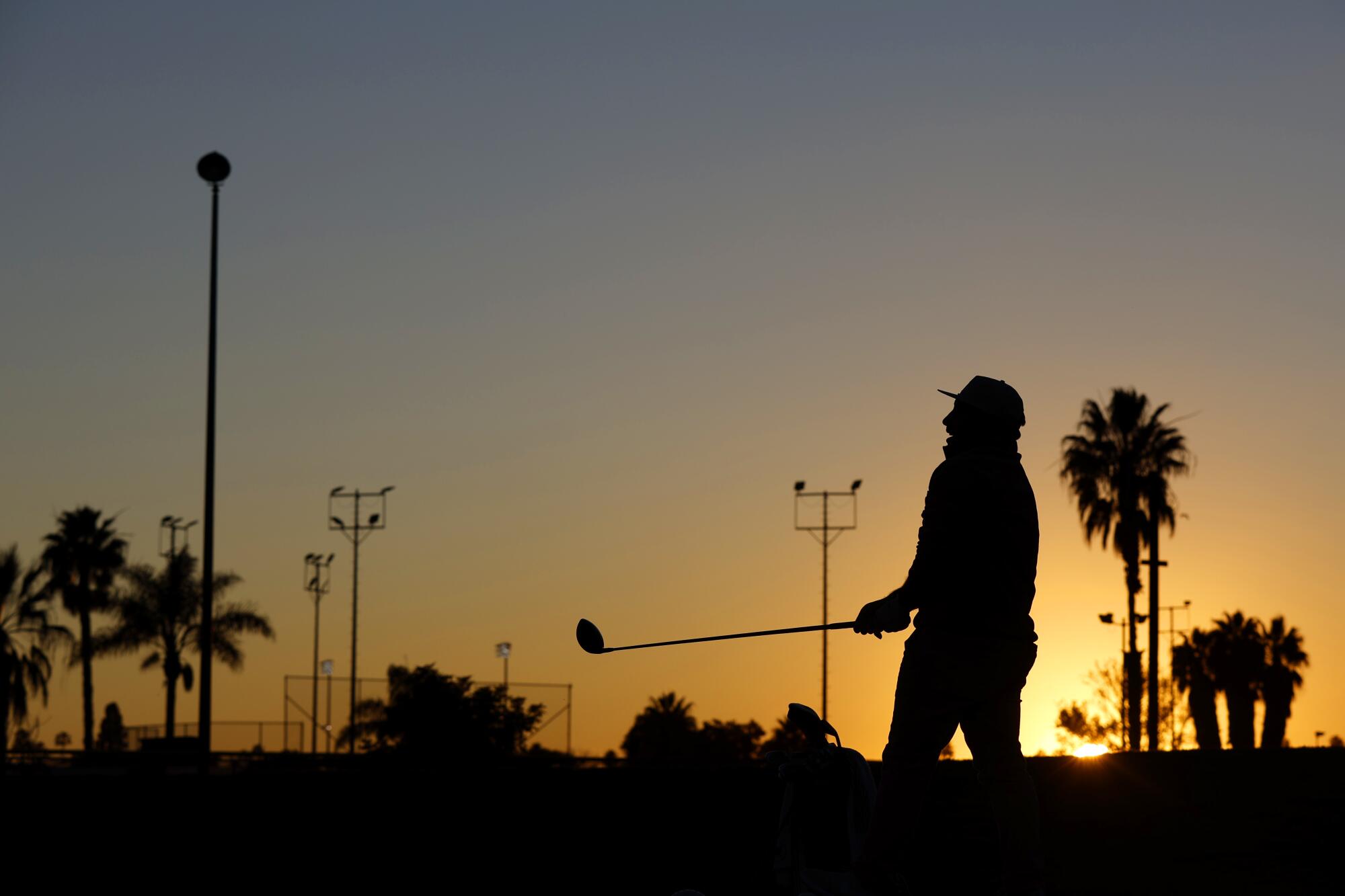Under the glow of a setting sun, a silhouetted man stands poised on a golf course, captured in mid-swing. The sky above transitions from a deep grayish-blue at the top to an expanse of warm yellow closer to the horizon, where the sun is just beginning to sink. The lower sixth of the image is dark, almost black, marking the ground and the distant horizon. The man, facing left, holds a golf club aloft with both hands, his head turned upwards to follow the trajectory of his shot. His expression, though subtle in the silhouette, hints at a sense of satisfaction or interest. He wears a forward-facing baseball cap, a long-sleeved shirt or jacket, and golf pants. Several palm trees and tall light poles, possibly around a baseball field, dot the distant background, adding to the tranquil yet dynamic ambiance of the scene.